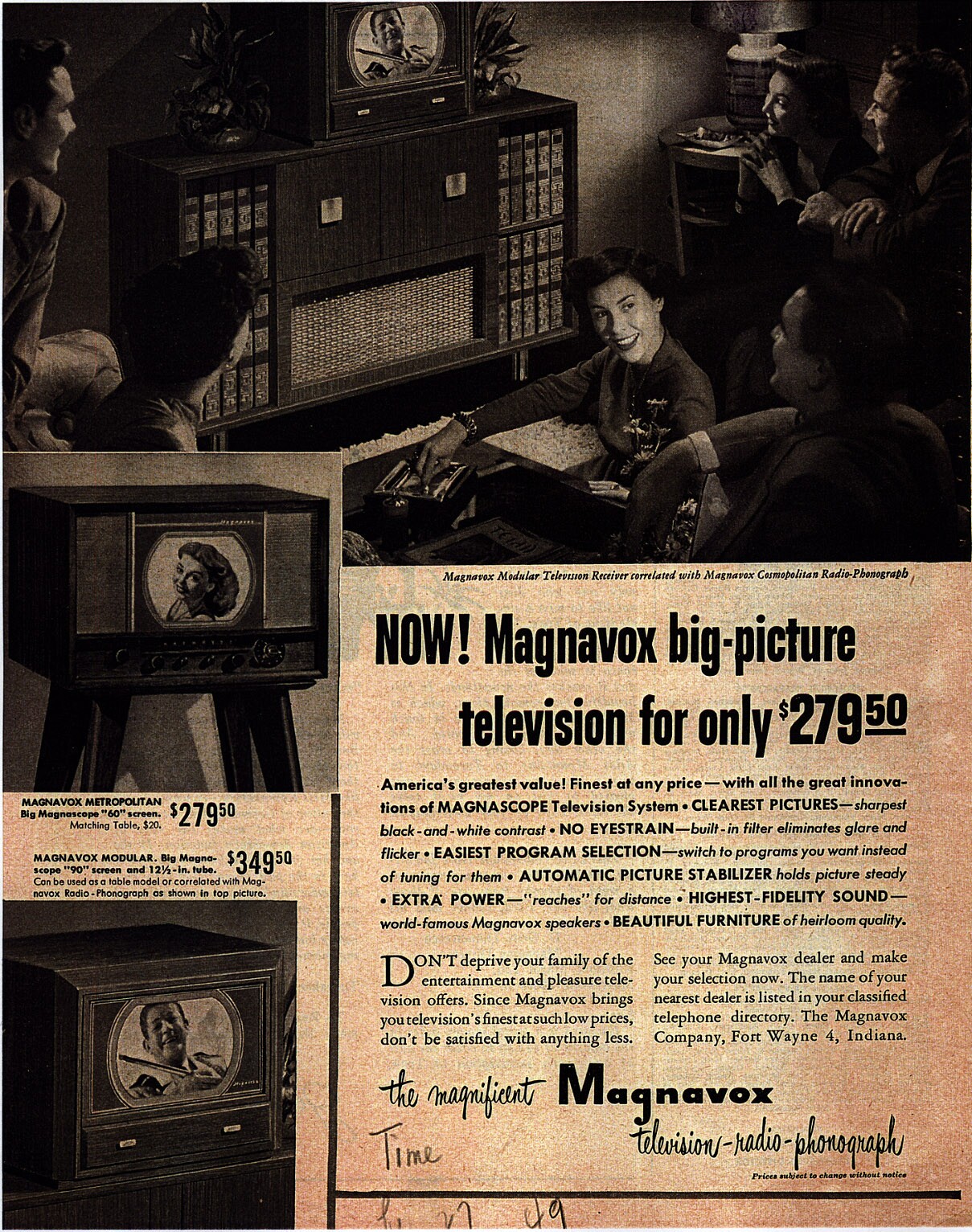The advertisement, a vintage piece likely from the 1950s or 1960s, showcases several Magnavox televisions in a nostalgic setting. At the top of the image, there is a warmly illustrated group of people gathered around a small TV with legs, evoking a sense of family and communal entertainment. This TV, referred to as the Magnavox Metropolitan, is priced at $279.50. Below this scene, on the left, is another image of the same TV model followed by its caption. Adjacent to this, you'll find a picture of the Magnavox Modular, a cubic TV priced at $349.50. Prominently positioned at the bottom right corner, bold text announces, "Now, Magnavox Big Picture Television for only $279.00." The advertisement extols the television's superior features, such as the MagnaScope television system's clear and sharp picture, anti-glare filter, automatic picture stabilizer, and world-famous Magnavox speakers. It emphasizes the high fidelity sound and the beautiful, heirloom-quality furniture design, urging customers not to deprive their families of the immense entertainment value. Further, the ad encourages readers to visit their local Magnavox dealer, with contact details available in the classified telephone directory.